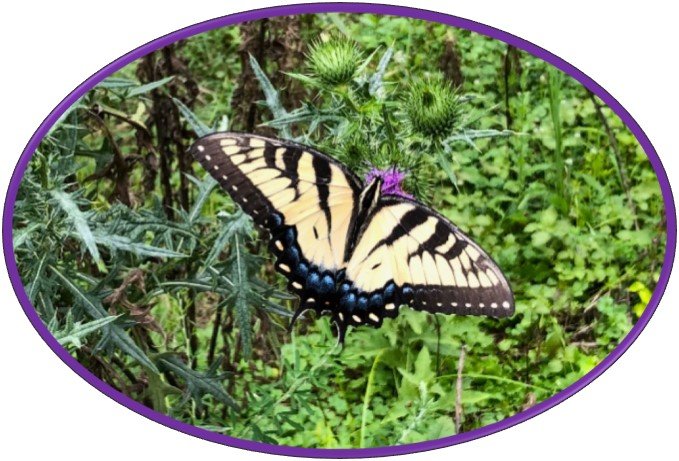The image showcases a close-up photograph, encapsulated within an oval frame with a thin, purple edge, set against a white background. At the heart of the photograph, a vivid scene unfolds: a beautiful butterfly is perched on a single purple flower, amidst an array of greenery that includes plants, trees, and bushes, suggestive of a forest setting. The butterfly, with wings fully spread, displays a striking coloration: primarily yellow wings adorned with black stripes, black edges, and accented with blue and yellow dots along its tail. The butterfly's back is notably yellow with a prominent black stripe. The detailed and realistic depiction of the butterfly, combined with the lush green background, makes it stand out almost three-dimensionally, enhancing the overall visual appeal of this serene natural moment.